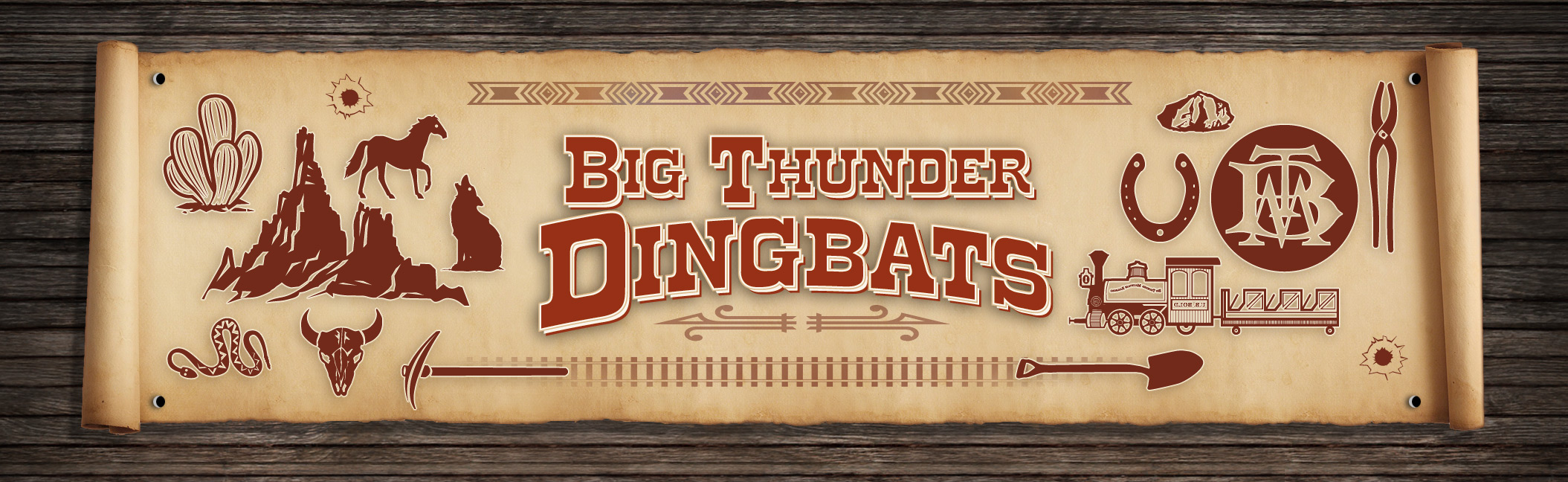In this detailed illustration, a metal sign or poster is shown, designed to look like it has been pinned or nailed to a thin, wooden panel wall. The sign appears slightly worn, resembling old parchment, but the imagery remains crisp. The background is a light beige, giving it an outdated, yet charming feel.

Prominently in the center, the sign reads "Big Thunder Dingbats" in a bold, dark red font. Surrounding this text are various dark red icons and symbols that add depth to the visual narrative. On the left side, there is a sequence of icons including a cactus, a mountain, a horse, a coyote, a sun, a Brahma bull's head, and a snake. These evocative images suggest a western theme. 

Below these icons, on the left, there is a pickaxe and a railway track, emphasizing the rugged and historic frontier life. On the right side of the sign, there are more icons, including a shovel placed below a depiction of the sun with a red center. Above the sun icon is an illustration of a train station or train, with red detailing on the front part and the car. Topping this visual ensemble is a red horseshoe, next to a symbol marked with the initials "BTM" in white lettering inside a red circle.

Further to the right of the sign are additional icons such as a pair of pliers and another depiction of a mountain. The detailed composition of the images, combined with the antique effect of the sign, may suggest it is an advertisement or a promotional piece, possibly for a musical group or entertainment troupe, adding a layer of intrigue and history to the scene.